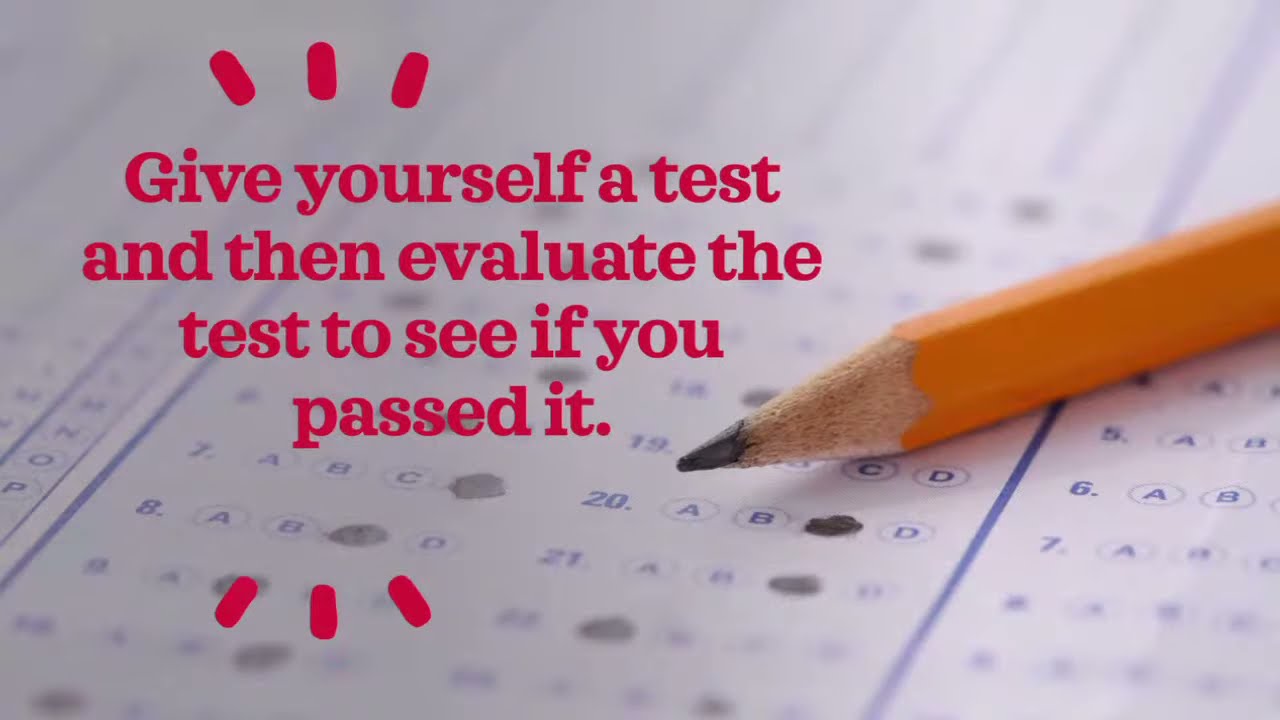The image prominently features a traditional fill-in-the-bubble answer sheet, reminiscent of Scantron forms used for exams. Lying diagonally across the sheet is a sharpened, standard number two pencil with an orange shaft, revealing only its graphite tip and a small portion of the body. Some of the test bubbles on the sheet have been filled in, showing selections of A, B, C, and D. On the top left corner of the image, vibrant red text in a bold serif font reads, "Give yourself a test and then evaluate the test to see if you passed it." Surrounding the text are small emanating lines, three at the top and three at the bottom, adding a sense of excitement and emphasis to the message. The combination of the traditional test sheet, the classic pencil, and the striking red text creates a nostalgic yet motivating visual, encouraging self-assessment and reflection.